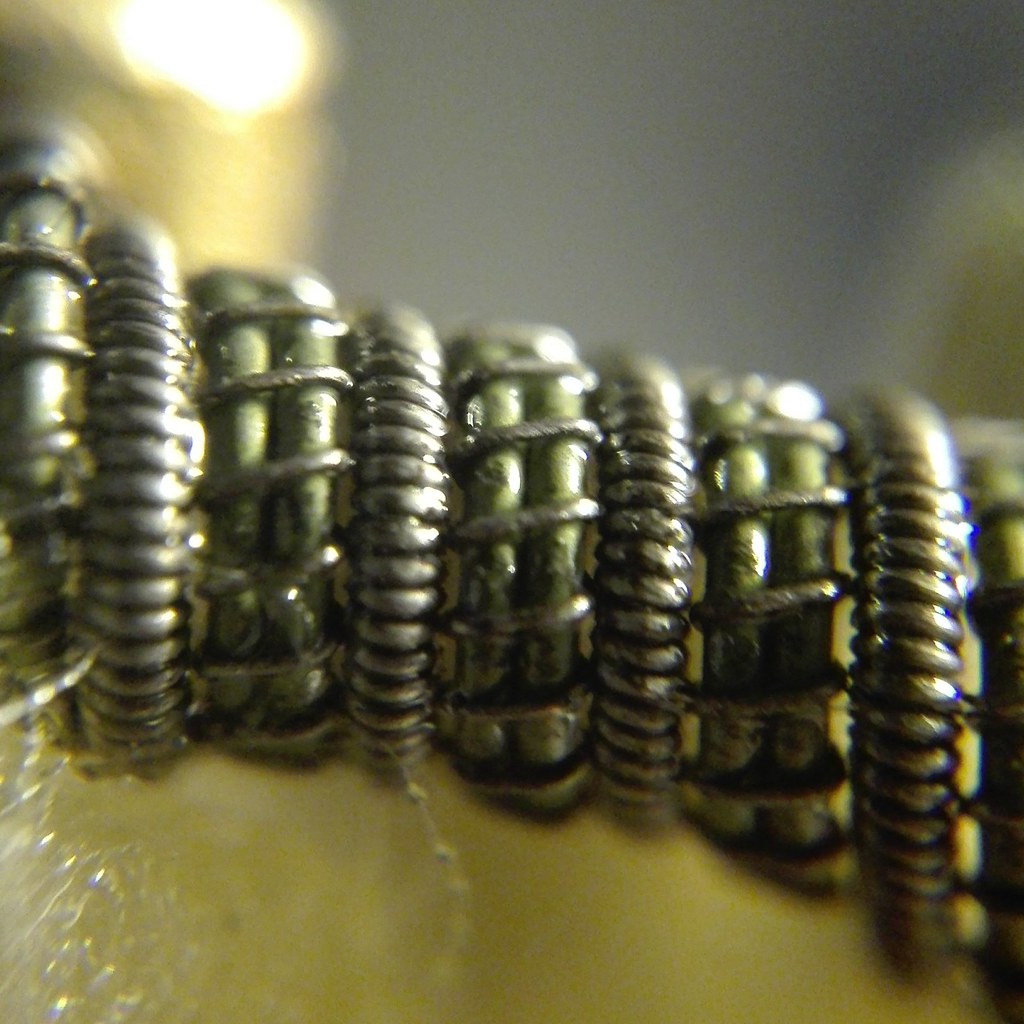This image is an extreme close-up, square format color photo of a metallic structure, possibly part of a bracelet or necklace, showcasing a detailed arrangement of wires. The object features alternating sections of two thick, brass-colored wires placed side by side, wrapped loosely by a thinner wire in a lateral looping pattern. Adjacent to these sections are tightly coiled, spring-like wires. This alternating pattern of loose and tight coils continues across the entire frame. The background is blurred, featuring dark gray hues with some golden tones. There is a noticeable reflection in the bottom left, suggesting the photo might have been taken through glass. Additionally, at the bottom of the image, there appears to be water leaking from the structure, hinting that it could also be part of a hose or tube, though the exact context of the object remains unclear.